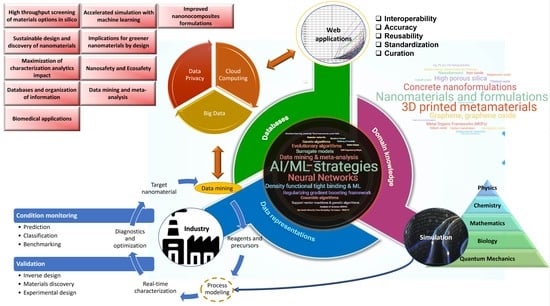The image is a detailed chart and diagram, possibly an information poster, showcasing AI/ML strategies and neural networks. In the upper left corner, there are nine pink rectangles with black text, aligned in three columns: three in the top row, two directly below, another two beneath, and the final two at the bottom. Below these rectangles on the far right, there is a circle divided into three sections with white text. An arrow points back and forth from this circle to another white circle above and to the right, which contains black text. To the right of this white circle, there are five lines of black text, each seemingly a single, unreadable word. 

Below the second white circle, a green band moves downward and leftward, forming part of another circular image divided into green, blue, and purple sections. Inside this colorful circle is a black circle with the prominent text "AI/ML Strategies" in white. To the right of this black circle is a smaller black circle and a green triangle, both containing unreadable text. To its left is a small white circle depicting a couple of buildings and some black writing. 

In the bottom left-hand corner, there are two thin blue rectangles with white text and black text beneath them. The middle right side of the image features faint lines with small text at the top, followed by the words "CONCRETE something" in red letters. Below this are the phrases "nanomaterials and formulations" in light green letters and "3D printed metamaterials" in red, with very small writing beneath that. The overall presentation includes various charts and diagrams, emphasizing AI/ML strategies, neural networks, domain knowledge in pink, data organization in blue, databases in green, and numerous subheadings and detailed notations.